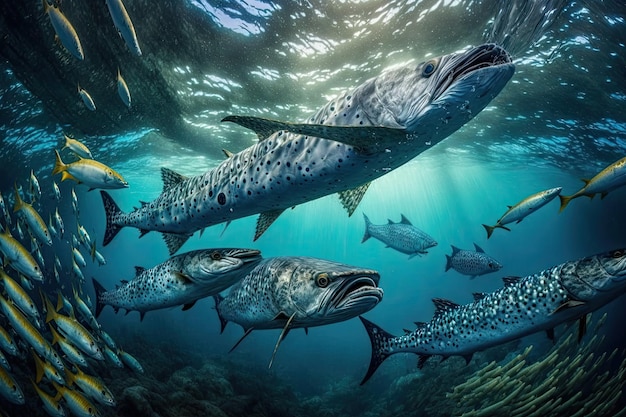This stylistic underwater artwork captures a vibrant marine scene teeming with life. At the top of the frame, the mottled undersurface of the water reveals a tapestry of black, white, and lighter blue streaks, illuminated by beams of golden sunlight filtering through. The pale blue water transitions through a gradient into a darker blue arc, culminating in a brownish-gray seabed at the very bottom. 

Dominating the scene are large, elongated fish, possibly barracudas, characterized by their open mouths, black eyes, mottled gray fins, and bodies adorned with black dots on their silver scales. The largest fish is centrally positioned with two smaller ones beneath it, and another similar fish is in the bottom right corner, partially cut off. 

Complementing the larger fish are schools of slender, smaller fish. In the bottom left, a school angles downward, each bearing silver bellies and yellow tops with yellow fins. Additional schools can be seen swirling around the scene, with some fish near the top left and others emerging from the bottom and behind the larger fish. The intricate interplay of sunlight and water enhances the vivid colors and dynamic movement within this aquatic tableau, celebrating the diversity of marine life in a captivating and detailed composition.